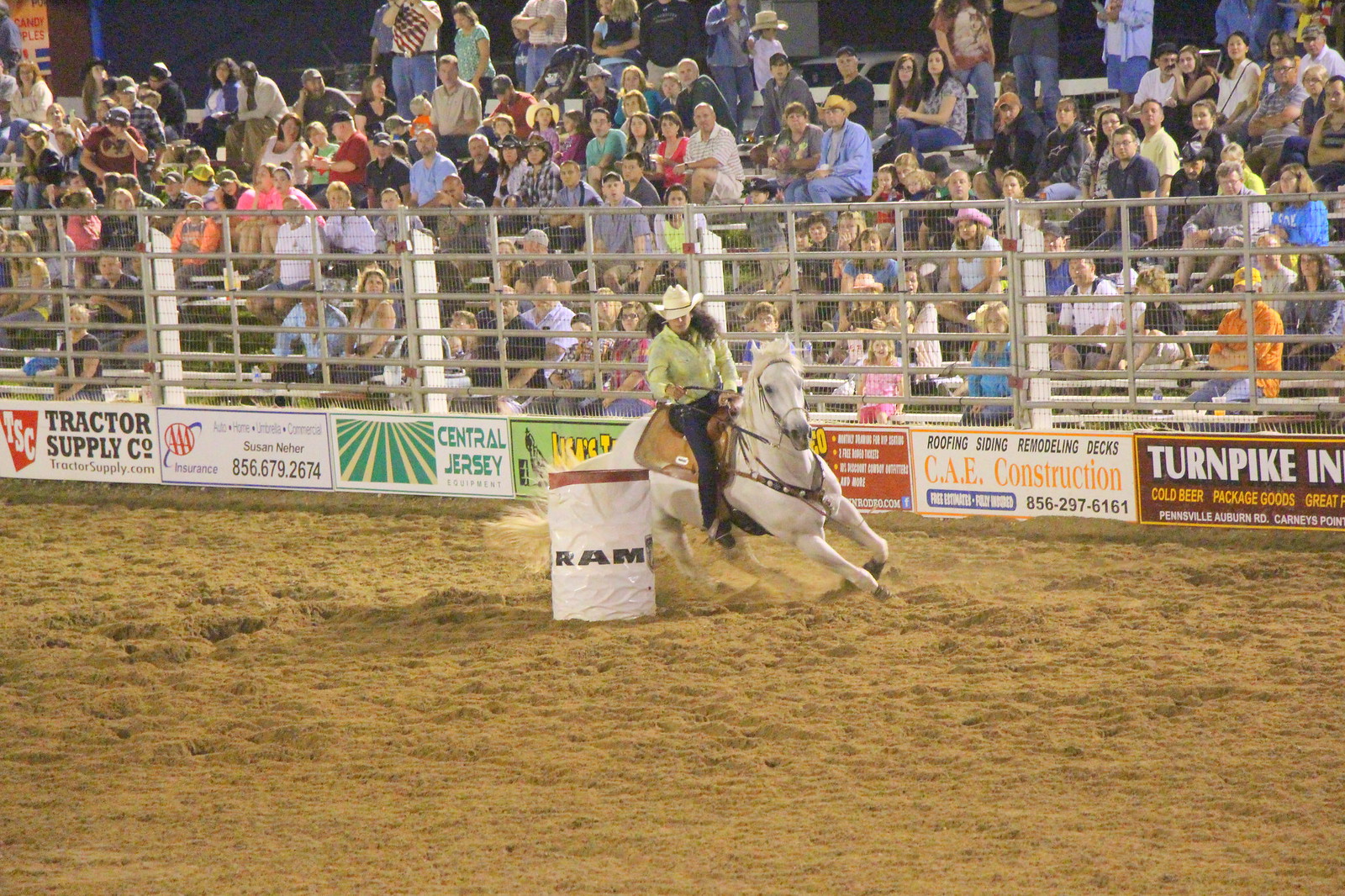In this dynamic image captured inside a dusty arena, a young woman clad in a light green button-up shirt, dark blue jeans, and a white cowboy hat is expertly maneuvering her almost-white gray horse around a barrel, which bears an advertisement for Dodge Ram. The horse, adorned in a western saddle and tack, leans sharply into the turn, showcasing the intensity of the barrel racing competition. Surrounding the arena, a tall, connected metal fence covered in advertisements from sponsors like Tractor Supply, AAA, Central Jersey, Turnpike Industrial, and K.E. Construction separates the track from a packed audience. The bleachers rise about ten rows high with spectators donning various attire including cowboy hats, baseball caps, shorts, and jeans, all avidly watching the thrilling race unfold in the brown, dusty confines of the arena.